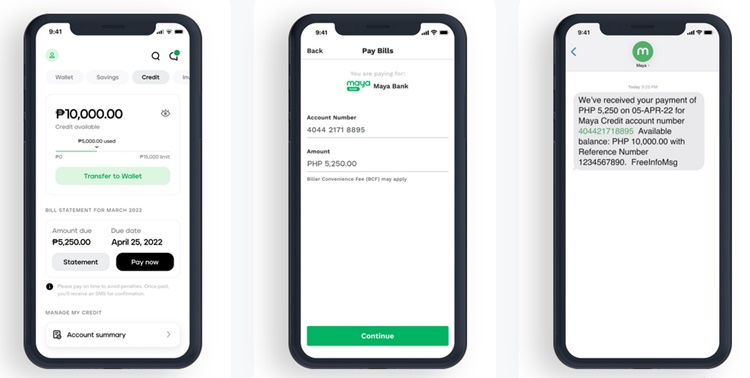The image series comprises three screenshots detailing a banking transaction, likely a bill payment. 

The first screenshot displays an account summary screen with options labeled 'Wallet,' 'Savings,' 'Credit,' and an obscured fourth option; the 'Credit' option is selected. The screen shows a credit balance of PHP 10,000 and mentions an amount due of PHP 5,250 with a due date of April 25th. The user has the option to pay this amount immediately. The account summary is provided at the bottom of the screen.

The second screenshot transitions to a payment interface for "Maya Bank," displaying the account number '4044-2171-8895.' It lists the payment amount as PHP 5,250 and has a 'Continue' button at the bottom.

The third screenshot confirms the transaction, indicating that a payment of PHP 5,250 was received on April 5th, 2022, for the Maya credit account matching the previously mentioned number. It also confirms the available balance as PHP 10,000 and provides a reference number for the transaction.